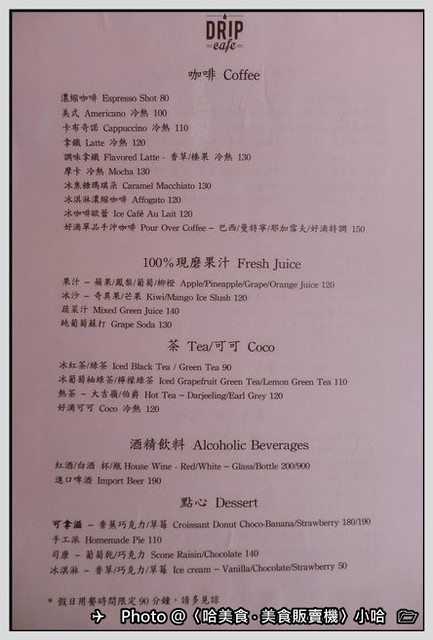This photograph showcases a legibly printed menu on standard-sized white paper (8.5" x 11"), featuring black text. At the top of the menu, the establishment's name, "Drip Cafe," is prominently displayed, accompanied by a graphic of a water or coffee droplet with a horizontal line extending from it. Below the café's name are Asian characters followed by the word "coffee."

The menu is organized into several sections. The first section lists coffee options, each entry featuring Asian characters, an English translation, and a price. For example, "Espresso Shot" is listed with the price "80." This format continues consistently for the rest of the coffee items.

Following the coffee section is a list of fresh juices, similarly detailed with translations and prices. Next, teas and cocoa are listed in their respective section. After that, a selection of alcoholic beverages is outlined. The final section at the bottom of the menu is dedicated to desserts.

Additionally, there is a white type print superimposed on the menu, featuring a small photo of an airplane. Below the airplane image, the phrase "photo at" is printed, followed by a series of Asian characters. This suggests that the image may have been a screenshot taken from a computer.